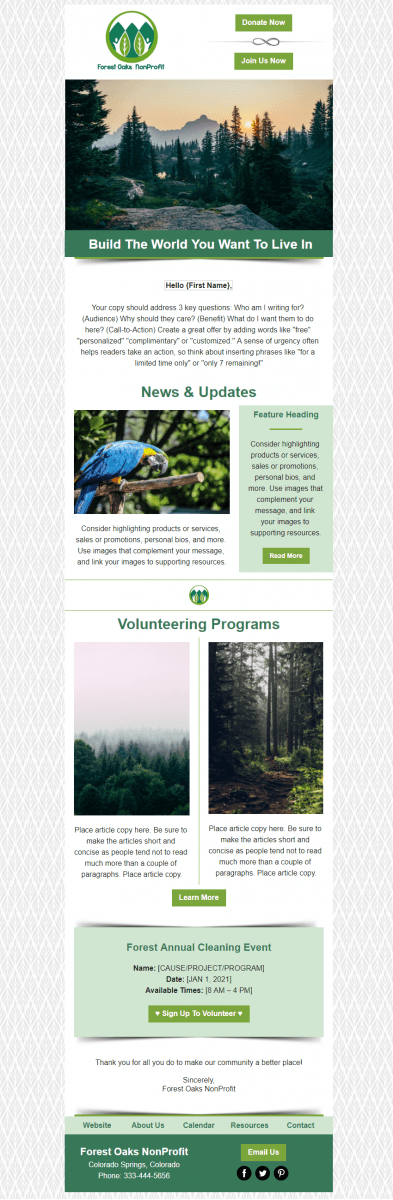The image appears to be a screenshot from a computer, featuring a long, narrow vertical layout. At the top, in green text, it reads "Forest [something] for Profit," though the exact wording is unclear. This header is accompanied by an image of leaves or trees. 

Beneath this, there is a captivating picture showcasing a mountain landscape at sunset, framed by trees, with the inspirational phrase, "Build the world you want to live in" displayed prominently.

Following this section, a greeting reads "Hello," with a placeholder for a first name in parentheses, suggesting personalized content might follow here. A section titled "News and Updates" in green text features a vibrant image of a blue and yellow parrot perched on a tree.

Further down, another heading reads "Volunteering Programs," accompanied by two images: one depicting a white sky over a tree-filled forest, and the other providing an immersive view of dense forest vegetation. 

A green "Learn More" button is centrally located for navigation. Below this button, a green rectangle announces the "Forest Annual Cleaning Event" with a specified date.

At the very bottom of the screenshot, in a green bar, the text reads "Forest Oaks Non-profit," followed by an invitation to email the organization.